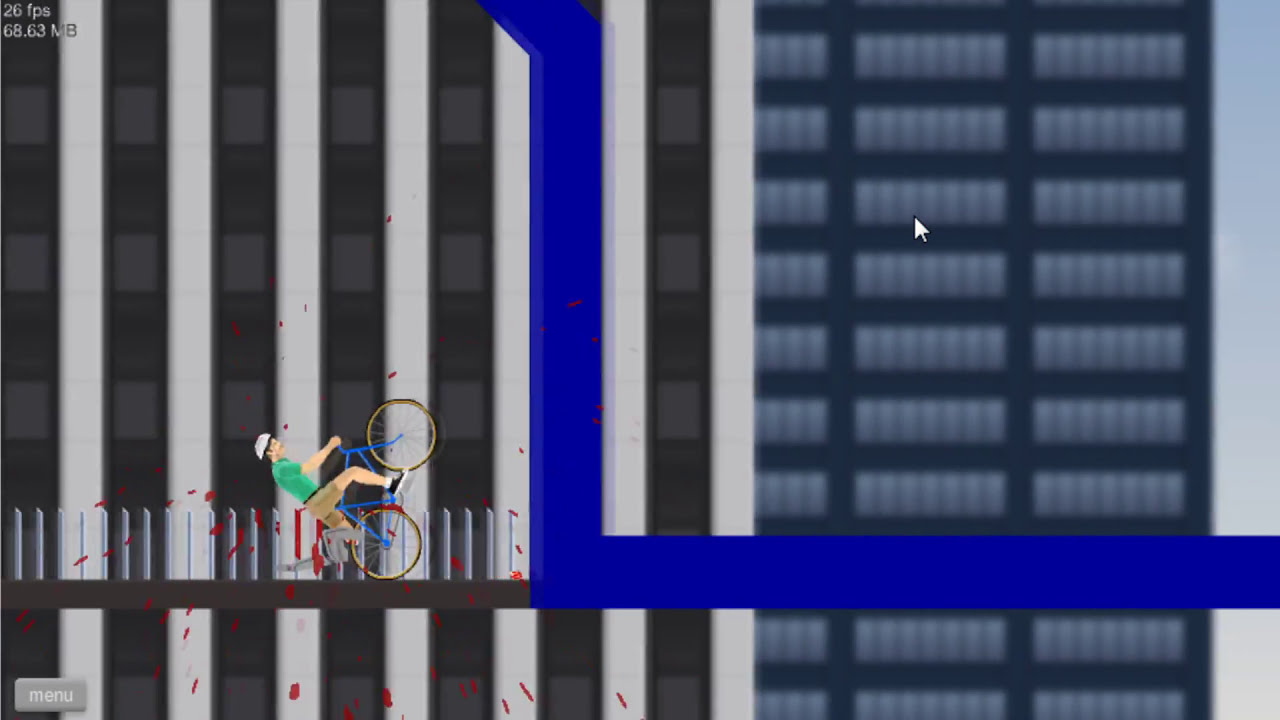This image is a still frame of a two-dimensional side-scroller video game. In the top left corner, white text shows "26 FPS" with "68.63 MB" just below it. The scene prominently features a city landscape backdrop with tall skyscrapers. Dominating the center is a blue line that descends and sharply turns right, leading off the screen. A gray menu button labeled "menu" in white resides in the bottom left corner. The focus is on a character riding a bicycle from left to right, though he appears to have fallen onto a series of tall silver spikes. Blood splatters around him as he leans far back, wearing a green shirt, white helmet, brown shorts, and black shoes. The building in the background has evenly spaced sets of windows framed by black strips and columns, contributing to the urban setting of the game.